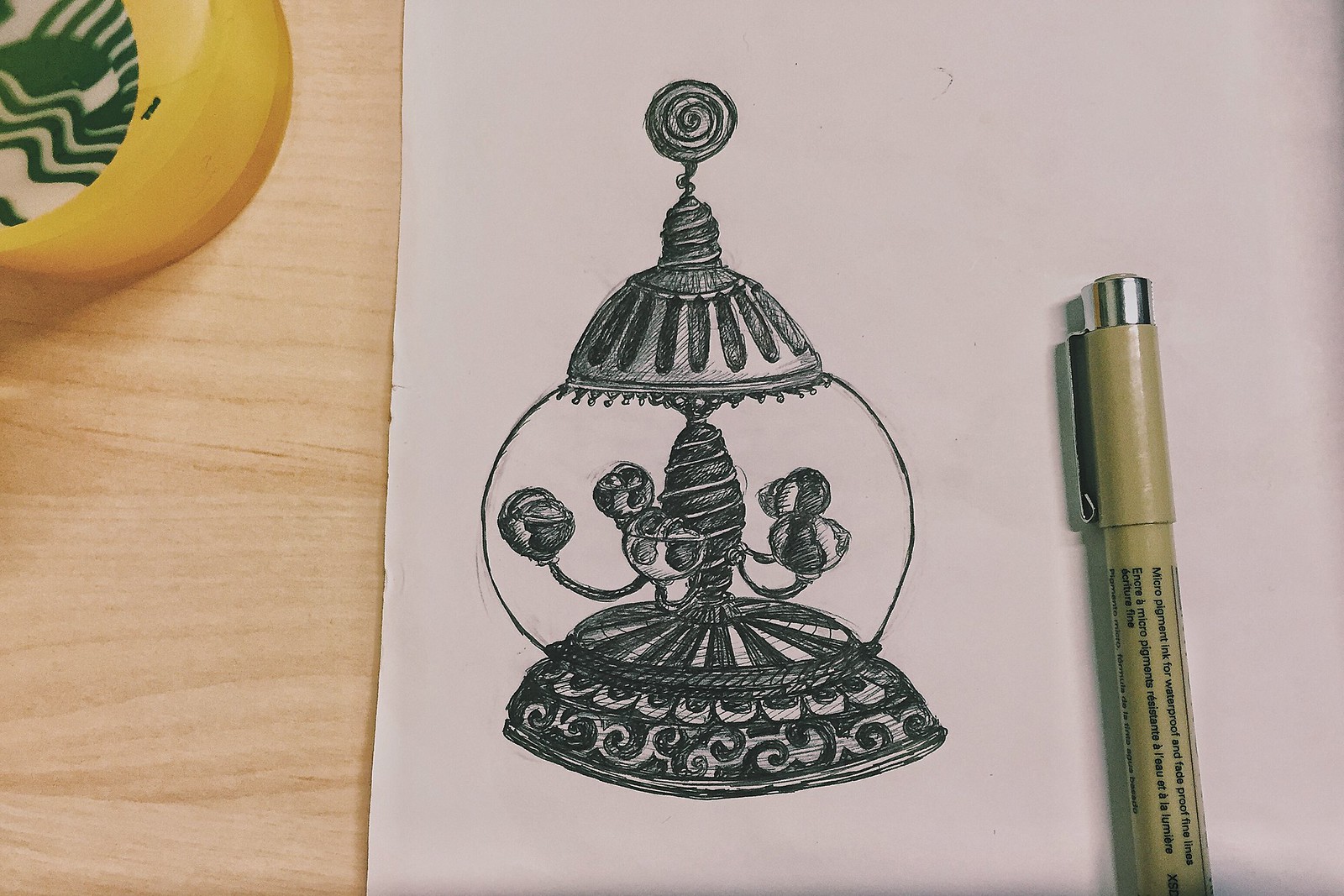In this monochromatic drawing, depicted on a white sheet of paper, a globe-like object resembling a snow globe catches the eye. Crafted with black ink or pencil, the circular globe features a simple black outline. Within the confines of the sphere, a whimsical carousel structure is present, reminiscent of those seen at carnivals. This carousel showcases globe-like planets orbiting a central axis. The globe's top is capped with a dome, crowned by a spiraling cap that culminates in a lollipop-style spiral design. The base of the globe displays an intricate geometric pattern, combining wavy and spiral elements colored in black with interspersed white spaces.

Surrounding the drawing, the white paper starkly contrasts with its content. The scene is set upon a light brown wooden table or desk. On the top left corner, a yellow plastic cup bearing a green Starbucks logo partially overlaps with the paper. At the bottom right of the image, half of the drawing instrument is visible; it is a tan cylindrical pen or pencil with a silver end cap. This detailed composition integrates everyday objects with imaginative artistry, creating an intriguing visual narrative.